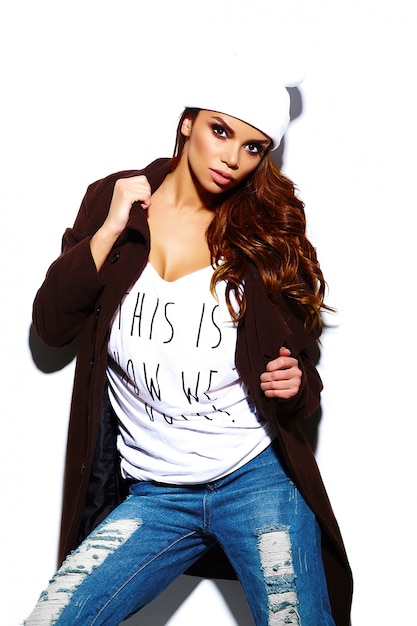This image showcases a woman modeling a stylish outfit against a white background. She is facing the camera with her head slightly tilted to her left, her long, wavy brown hair cascading over her left shoulder. She is adorned in a snug white beanie hat and sporting a meticulous makeup look with a tanned complexion. Her expression is neutral as she looks slightly down toward the camera.

The woman is dressed in a dark brown long-sleeve coat that reaches down to her knees. She holds the coat's collar delicately with her right hand raised near her neck, while her left hand grasps the coat's side, her knuckles facing the camera. Beneath the coat, she wears a loose-fitting white shirt with black lettering that reads, "This is how we do it."

She completes her ensemble with a pair of blue denim jeans, which feature frayed details down the front, giving them a distressed, worn-in look. Her stance is poised and confident, with her legs slightly spread apart and her right leg subtly turned left. This finely orchestrated pose, combined with the absence of distracting elements, highlights the professional nature of the photograph.